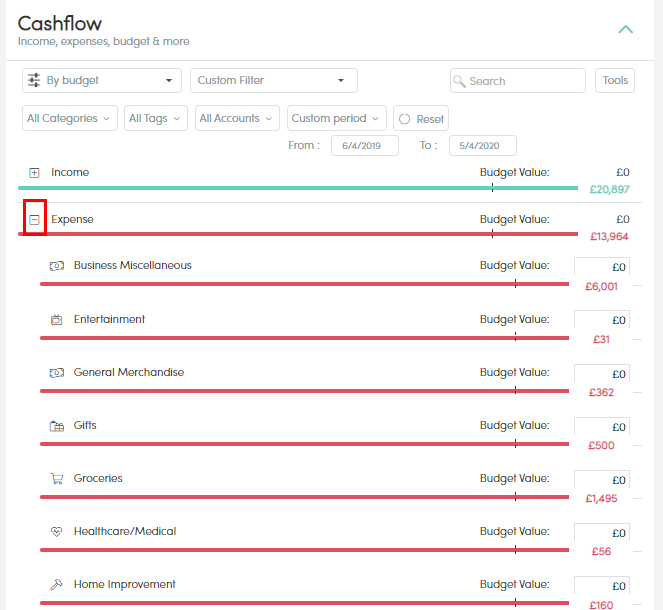This page provides a detailed financial overview and budget tracking for the period from June 4, 2019, to May 4, 2020. In the top left corner, there is a section dedicated to cash flow, alongside categories for income, expenses, and budget. Filter options are available at the top, allowing users to sort by budget, apply a custom filter, and view details across all categories, tags, and accounts.

The left column categorizes various financial aspects such as income, expenses, business expenditures, miscellaneous costs, entertainment, general merchandise, gifts, groceries, healthcare, medical expenses, and home improvements. Adjacent to each category on the right, the respective budget values are displayed.

For instance, the income is precisely calculated at £20,897, followed by another significant amount of £13,964. Each subsequent line item provides specific monetary values, ensuring a comprehensive and clear picture of the financial summary for the chosen time period.